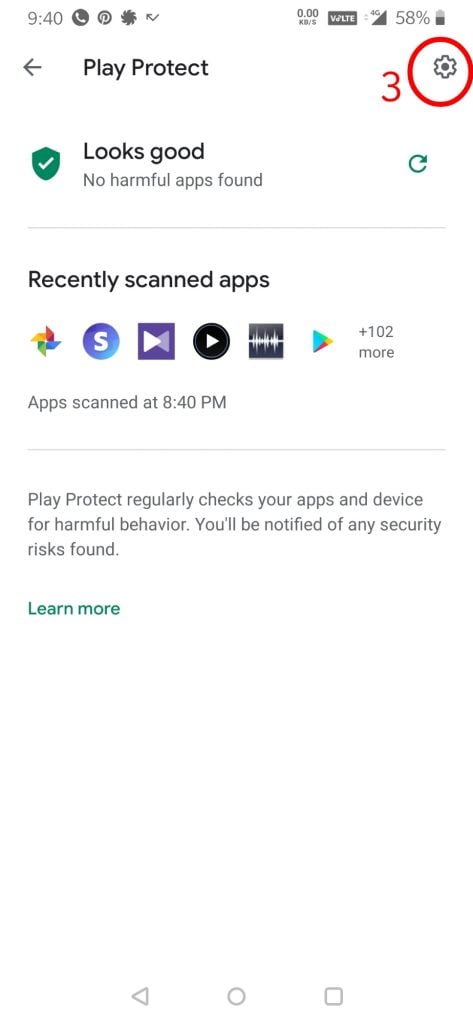A screenshot of a smartphone screen displaying various system notifications and statuses. At the top of the screen, the time is shown as 9:40. There are small symbols including a gray circle with a white phone icon, a Pinterest icon, and a couple more symbols: a star and a bent arrow curving down to the left and then up to the left. Adjacent to these symbols, some small text indicates "0.00" and the battery level, which is at 58%.

Beneath this, the screen features a notification from Google Play Protect, displayed in black text, stating "Play Protect." Accompanying this message is a left-pointing arrow. To the right, there is a red circle containing the number "3," which surrounds a settings icon. Directly subsequent is a green checkmark confirming "Looks good" and indicating that no harmful apps were found.

Further down, the notification lists "Recently scanned apps" with icons representing applications like Skype, Google Play, and Google. There is also a note indicating there are additional applications, with a plus sign and the text "+102 more."